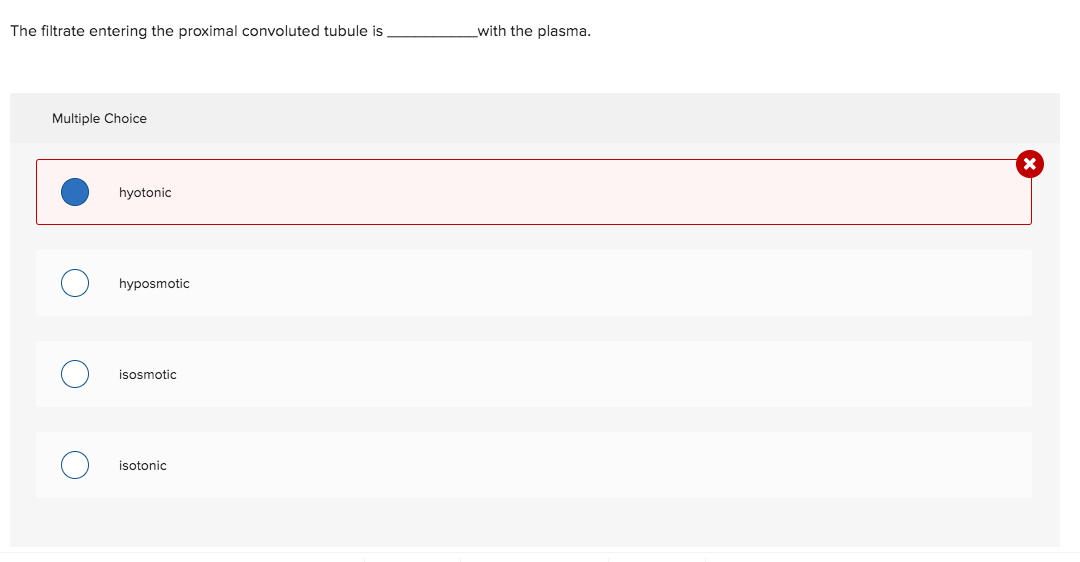In the image, a multiple-choice quiz question is displayed, asking about the nature of the filtrate entering the proximal convoluted tubule in relation to the plasma. The user had four options: hypotonic, hyposmotic, isosmotic, and isotonic. They selected 'hypotonic,' which is highlighted in red, indicating an incorrect choice. The entire multiple-choice area is set against a light gray background, with each answer option presented in a long, wide rectangle that features a selection bubble on the left side. The scene appears minimalistic, with no additional elements. The user speculates that a correct answer would be highlighted in green, possibly accompanied by a check mark. The overall design suggests that this image might have originated from a biochemistry or pre-medical course material.